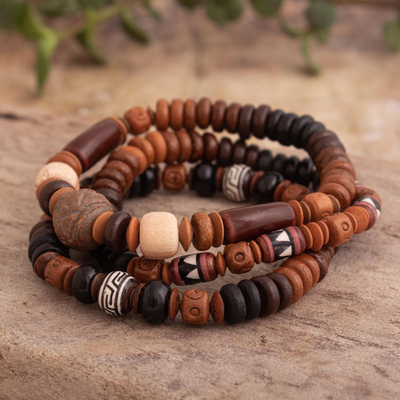The image captures a close-up of three distinct wooden bead bracelets arranged in a stack on a rustic, rough wooden surface. The bracelets, seemingly handmade, showcase a variety of bead shapes and sizes, including round, thin, thick, and square beads. Their color palette ranges primarily in hues of brown, dark brown, light brown, tan, black, and white. Notably, one bracelet features a bead with a white trim and intricate design, while another has white-trimmed beads adorned with triangles and some black and white squiggly lines. Each bracelet also includes elongated beads, adding to their unique, yet coordinated, appearance. In the blurred background, green plant foliage peeks through, enhancing the natural, earthy feel of the composition. It's a harmonious mix of textures and colors, highlighting the artisanal craftsmanship of these wooden accessories.